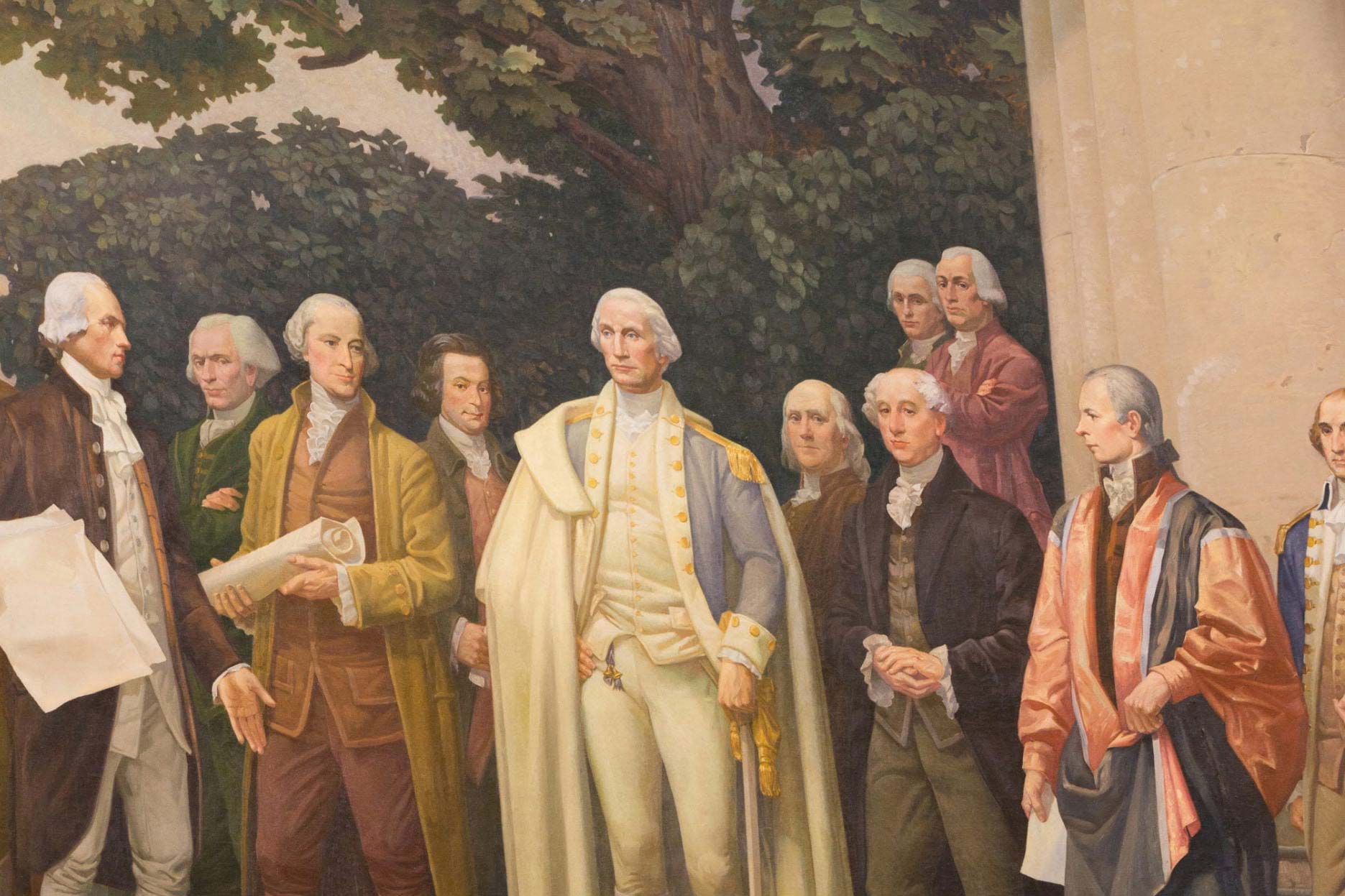This detailed color illustration, likely an old oil painting from the late 1700s or early 1800s, depicts a group of distinguished white men, possibly noblemen or statesmen from the early United States. Centered in the painting is a figure resembling George Washington, adorned in a blue military uniform with white cuffs and collar, a long white coat draped over his shoulders, and white pants. His left hand rests on the hilt of a sword, and he exudes a commanding presence. He is flanked by several other men, many of whom are wearing white wigs, signifying their period dress. To the immediate right of George Washington stands a figure resembling Benjamin Franklin, donning a green jacket.

To the left of Washington, there is a man in a brown jacket holding a large piece of paper, and another in a yellow jacket with an orange-brown suit, both exhibiting skeptical or unhappy expressions. The figure on the far left, with a glaring expression and folded arms, stands out for his displeased demeanor. 

In the background, a large tree with a lush green canopy towers above the scene, complemented by a peach-colored wall on the right side of the image. The various gentlemen around Washington appear engaged, some seemingly skeptical or angry, adding to the painting's historical and atmospheric depth.